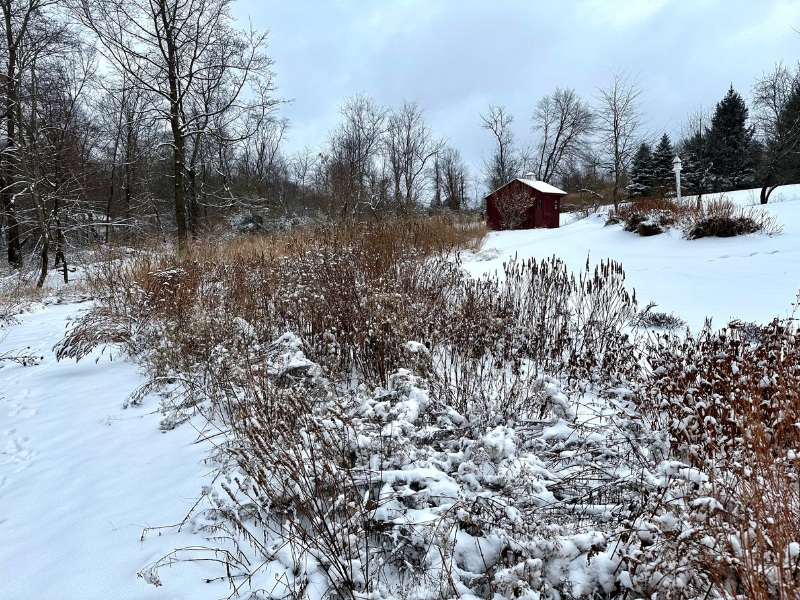The rectangular color photograph captures a serene winter scene on a hillside. In the foreground, a thicket of cattails and brown shrubbery, lightly dusted with three to four inches of snow, occupies the center. The snow-laden vegetation and minimal snow accumulation emphasize the wintry landscape. To the right, the photo reveals a more cleared area with patchy snow on the ground. 

Further back, nestled amidst this wintry meadow, stands a small structure—possibly a cabin or shed with a dark wooden or brownish-red exterior. The structure is partially obscured but identifiable by its snow-covered roof and small metal chimney. This building is one or two stories high and features a couple of windows, accentuating its rustic charm.

In the distant background, the scene is framed by barren trees with several evergreen trees visible in the upper right corner, some of which are capped with snow. The sky above is a typical winter grayish-blue, heavy with cloud cover, casting a soft, diffused light over the entire landscape. To the left of the image, faint footprints trace a path through the snow, leading towards the cabin, adding a subtle human touch to this tranquil winter panorama.